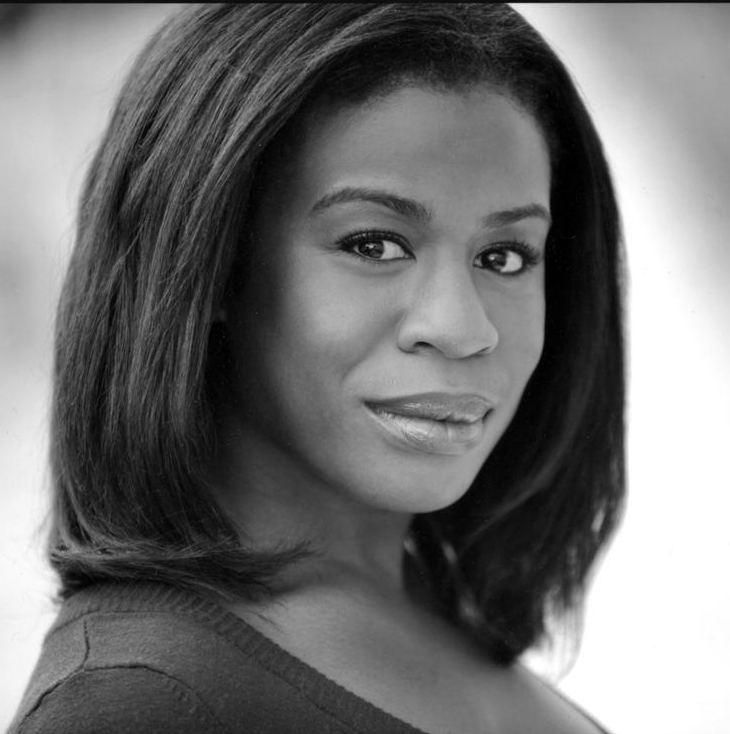This black and white image features a close-up of an African American woman with smooth, clear skin and expressive, dark eyes. Her long, thick black hair is straightened and falls just above her shoulders. She is wearing a dark-colored shirt with a threaded design around the shoulders, revealing a subtle glimpse of her chest. Her body is slightly turned to the right, but her face is directed towards the camera with a gentle, closed-mouth smile. The background of the photograph is blurry and predominantly white with hints of gray, suggesting the picture may have been taken outdoors.